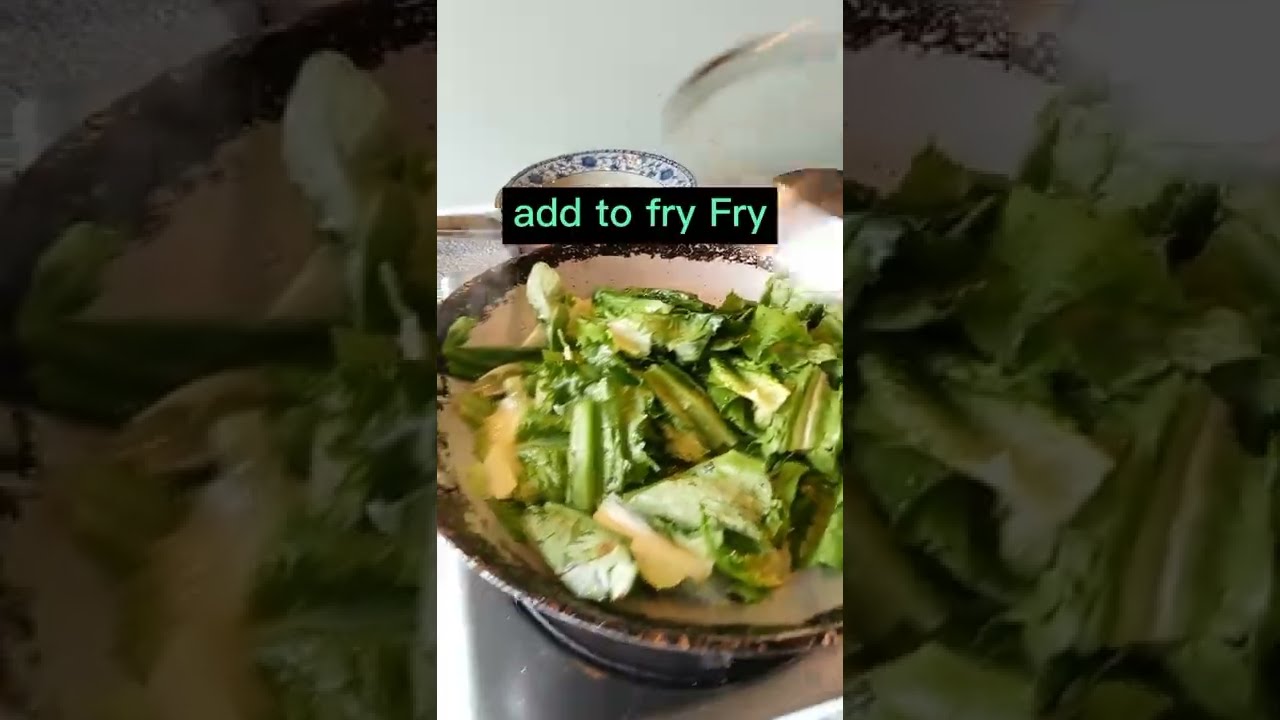The image features a vertical photo of a rustic salad bowl with a rough, black-painted rim and a white interior. Inside the bowl, there is a mix of roughly chopped green lettuce or kale, and possibly some pieces of cauliflower, lightly dressed with what appears to be a vinaigrette. Hovering over the bowl is a black caption box with teal text that awkwardly reads, "Add to Fry, Fry," with the second "Fry" oddly capitalized. In the background, another bowl with a white interior and a detailed China blue rim can be seen. The left and right sides of the main bowl are flanked by close-up snippets of the same image, creating a magnified, shadowed effect. This composition suggests a messy yet artistic presentation, giving a detailed and somewhat chaotic overview of the scene.